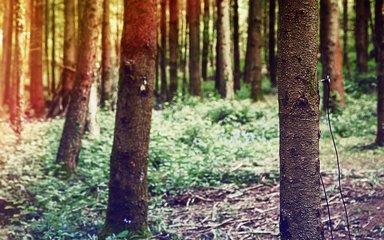This close-up forest photograph captures a serene scene where tree trunks dominate the view, rising from a ground carpeted with brown soil and green foliage. The trees, uniformly thin with dark brown bark, range from 5 to 10 inches in diameter, hinting at their mature yet not ancient age. The tree trunks are concentrated but sparse enough near the foreground to reveal patches of soil and vibrant green moss, particularly on the trunk closest to the camera. On the left side, golden sunlight filters through a dense grouping of trees, casting an orange-red hue and creating a beautiful glare captured by the camera lens. Meanwhile, the center of the image reveals a small clearing, further accentuated by the sunlight, which contrasts with the darker, shaded areas on the right. The entire scene is bathed in a natural glow, illustrating a tranquil forest bathed in warm daylight.